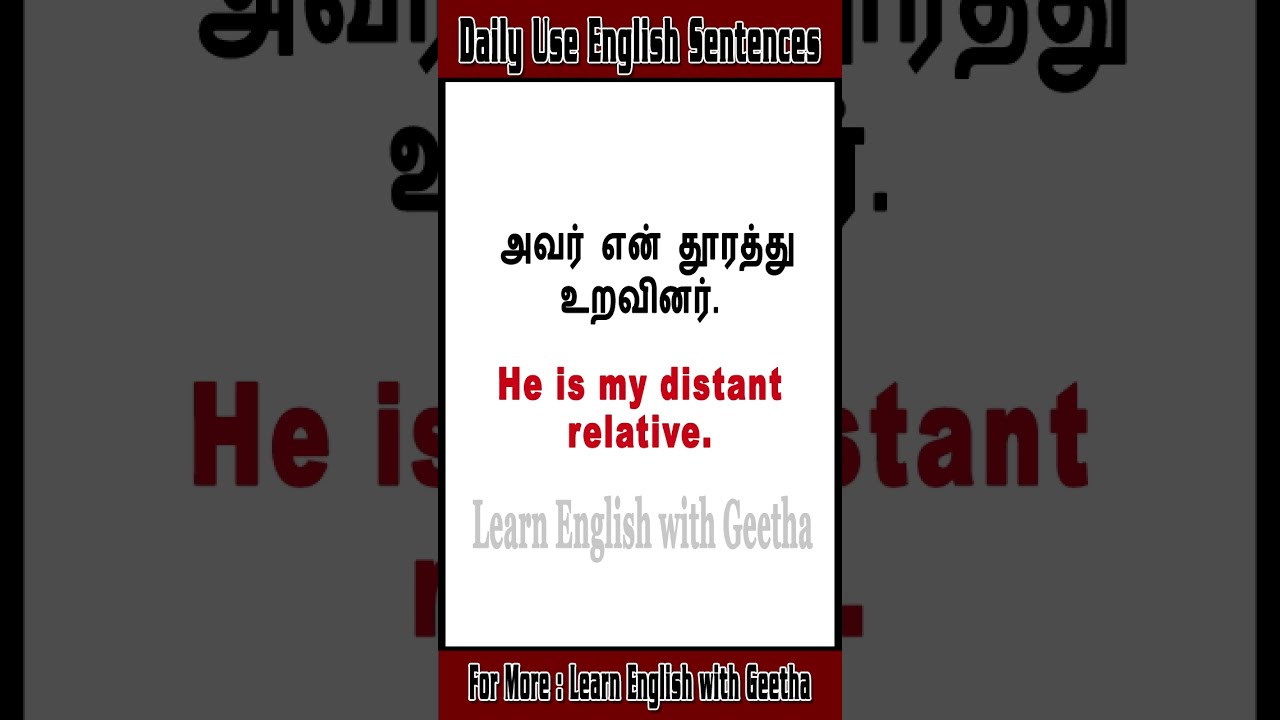The image is a promotional screenshot for a language learning app, presented in a vertical rectangle orientation, typically seen on mobile screens. The background of the rectangle is white with red borders at the top and bottom. Both borders feature black text outlined in white. The top red border reads, "Daily Use English Sentences," while the bottom red border states, "For more, learn English with Geetha, G-E-E-T-H-A." The central section of the image has a white background. At the top, there are two rows of black text in an indiscernible script that resembles Arabic or an Indian language such as Hindi or Tamil. Below this, there are two lines in bold red sans-serif font that read, "He is my distant relative." At the very bottom, in a very light gray serif font, it says, "Learn English with Geetha." The overall image suggests a still shot from a language learning channel or app, emphasizing the educational content available via Geetha. The primary colors used in the image are red, black, white, and gray.